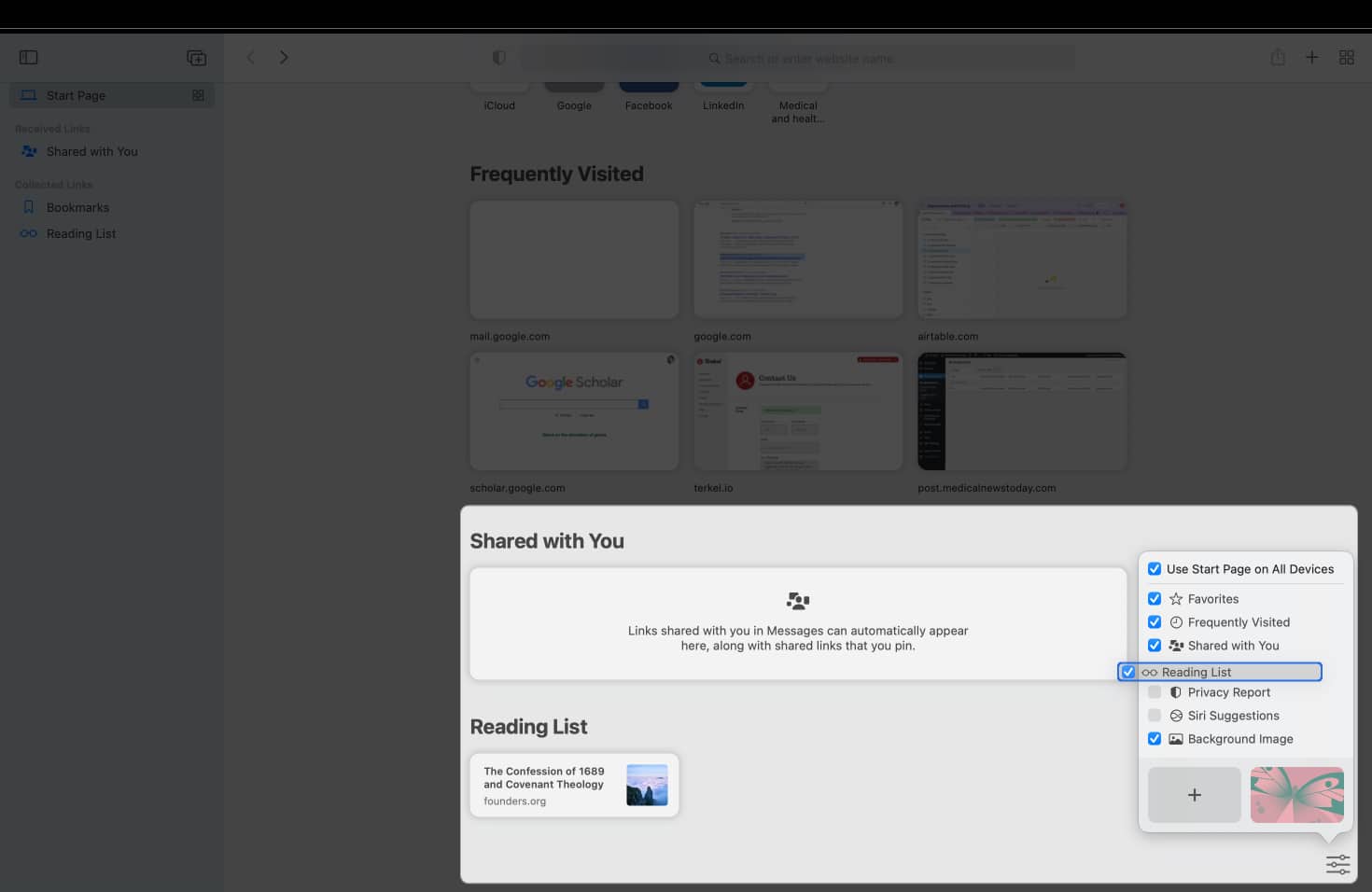This is a detailed screenshot from a computer displaying a customized homepage interface with a dark, grayed-out background. The main section features a series of frequently visited websites and categories including "Shared with You," "Start Page," "All Devices," "Favorites," "Frequently Visited," and "Shared." There is also an option for users to personalize this homepage.

The visual elements of the screenshot include a decorative butterfly graphic superimposed on the background. Below this image lies a series of suggestions and a reading list, which notably includes titles such as "Confessions of 1689" and "Covenant Theology." An area dedicated to bookmarks is also visible, showcasing a link to "Google Scholar."